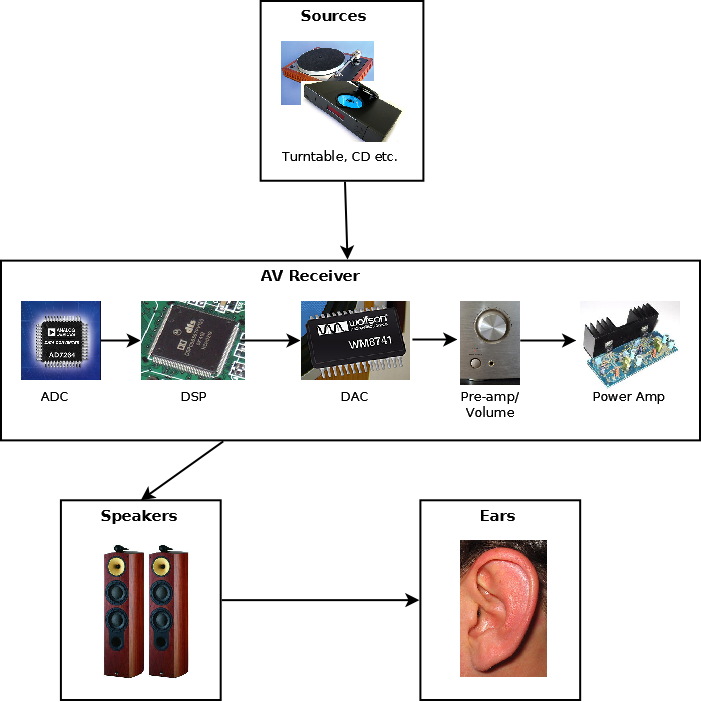This detailed diagram illustrates the path sound takes from its source to the human ear, featuring a series of images and annotated components. At the top, a labeled box titled "Sources" showcases a turntable and CD player, each finely detailed with descriptions; the turntable, housed in a wooden case, features a black circular top and a silver arm, while the adjacent CD player flaunts a blue CD and a red LCD screen. This "Sources" box directs an arrow to a larger rectangle named "A.V. Receiver," compartmentalizing its interior into smaller labeled images: an ADC chip (AD7284) with silver prongs, a DSP chip mounted on a circuit board, a DAC chip (WM8741) with elongated prongs, and a preamp/volume control unit depicted with knobs and a headset port. Following this sequence, next is an image of a power amplifier with a black heat shield and multi-colored transistors on a blue board. From the "A.V. Receiver," an arrow directs to a "Speakers" box displaying two tall speakers, a striking visual contrast of wood and varying cone colors and shapes. Another arrow links this to a concluding "Ears" box, featuring a close-up of a human ear with detailed skin tone and hair texture, representing the final destination of the sound path. This structured visual guide meticulously outlines how sound travels from its playback source, through various electronic components, to ultimately be perceived by the ear.